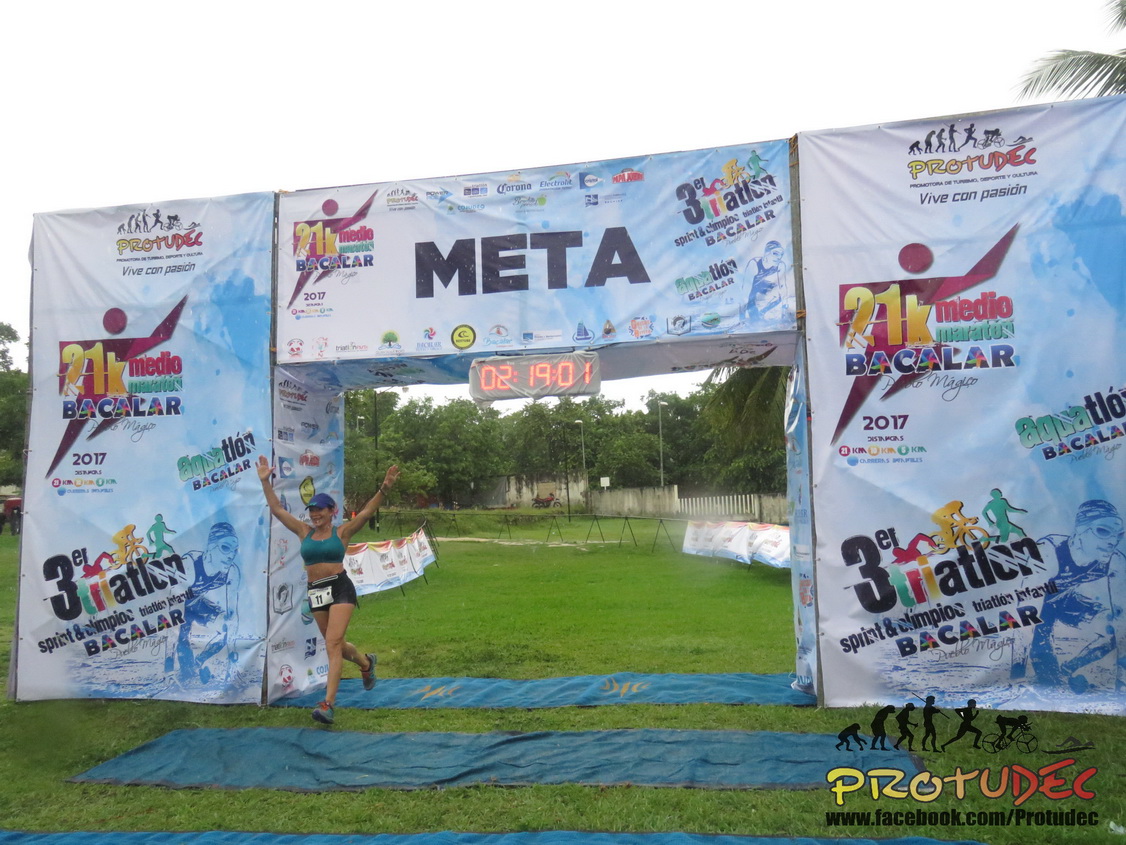The photograph captures the exhilarating moment at the finish line of a marathon. Framed by three metal structures adorned with banners, a female runner is triumphantly crossing under a large, square-shaped archway. The central structure prominently features an LED timer displaying "02:19:01" in bright orange numbers. The banners, consistent across the structures, are white with a blue graphic depicting someone emerging from water, along with numerous logos including one that reads "META," alongside others indicating "3 Triathlon," "Sprint," and "Olympic Barclay 2017."

The runner, positioned slightly to the center left of the image, sports a green sports bra, black shorts, and a blue visor. She has a white tag pinned to her shorts displaying the number "11" (or possibly "77") and raises her arms in celebration as she passes under the arch. Flanking the finish line are blue tarps, adding splashes of color to the scene. In the background, grassy fields are visible, demarcated by barriers guiding the marathoners' path. The image vividly captures the essence of completion and triumph, highlighting both the runner's achievement and the event's organized structure.